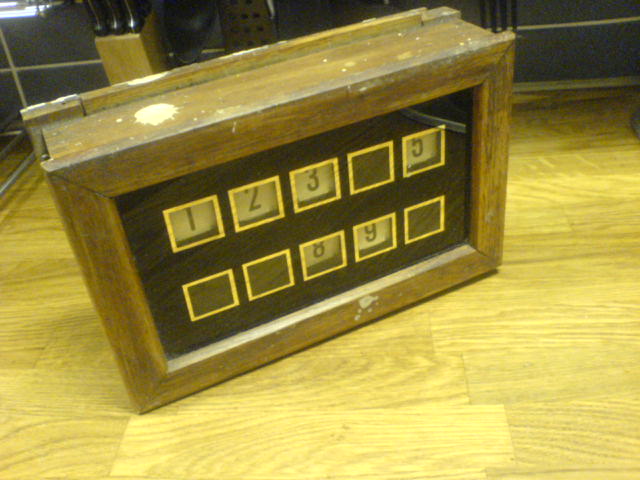The image features a wooden number box positioned at an angle on a light-colored wooden table. The box is robust and has a thick wooden frame with the center section slightly narrower but still substantial in thickness. There are noticeable paint drips on the top of the frame. The front of the box includes a glass face, underneath which is a black background adorned with ten small square cutouts, each bordered in gold. These cutouts display numbers on small white backgrounds with black text. The visible numbers are 1, 2, 3, 5, 8, and 9, while 4, 6, 7, and 10 are either blank or obscured. The number squares are slightly recessed, not flush with the glass. The table beneath the box has visible wood grains and wide planks, suggesting it's not of a farmhouse style due to its yellowish tint. In the background, there's a gray subway-tiled wall and a knife block in the upper left corner, contributing to the kitchen-like setting.